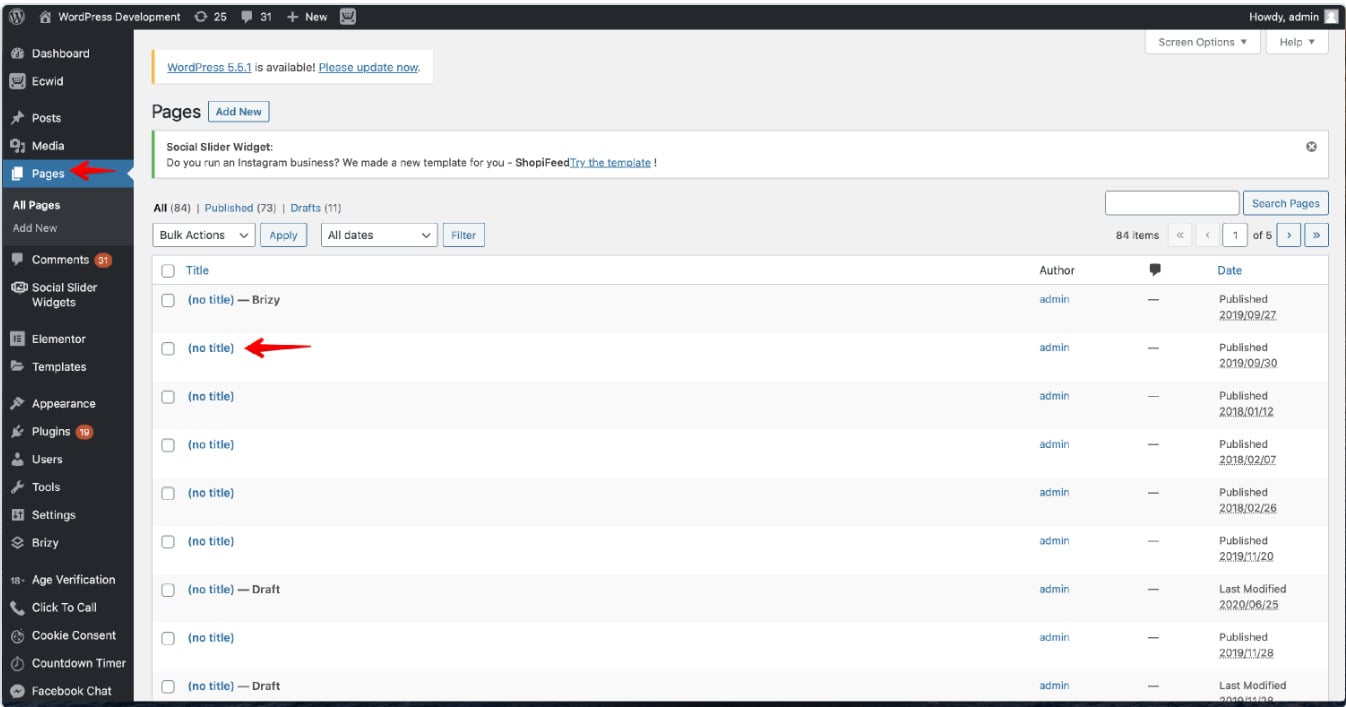Screenshot of a WordPress Admin Dashboard

The image captures the interface of a WordPress admin dashboard. At the top, a white notification banner highlights that "WordPress 5.5.1 is available" and prompts the user to "please update now." Adjacent to this banner is a vertical yellow line. Directly below, a blue button labeled "Pages, Add New" is prominently displayed.

A green vertical line traverses the section just beneath the banner, signaling a notification for a "Social Slider Widget." The widget message asks, "Do you run an Instagram business?" and introduces a new template called "Shopee feed," inviting users to try the template via a clickable blue link.

The screenshot features two digitally added red arrows. One arrow points to the phrase "no title" located centrally on the screen. The second arrow points to a black vertical sidebar on the left side of the screen, targeting the "Pages" section. This sidebar contains various administrative categories including "Dashboard," "Euclid," "Posts," "Media," and notably "Pages," which is expanded to show "All Pages" and "Add New." Further down, the sidebar indicates the existence of "Comments" with 31 unread comments and "Plugins" with 19 notifications, continuing through more menu options.

The meticulous arrangement of these elements offers a comprehensive view of the user's current administrative tasks and notifications within the WordPress dashboard.